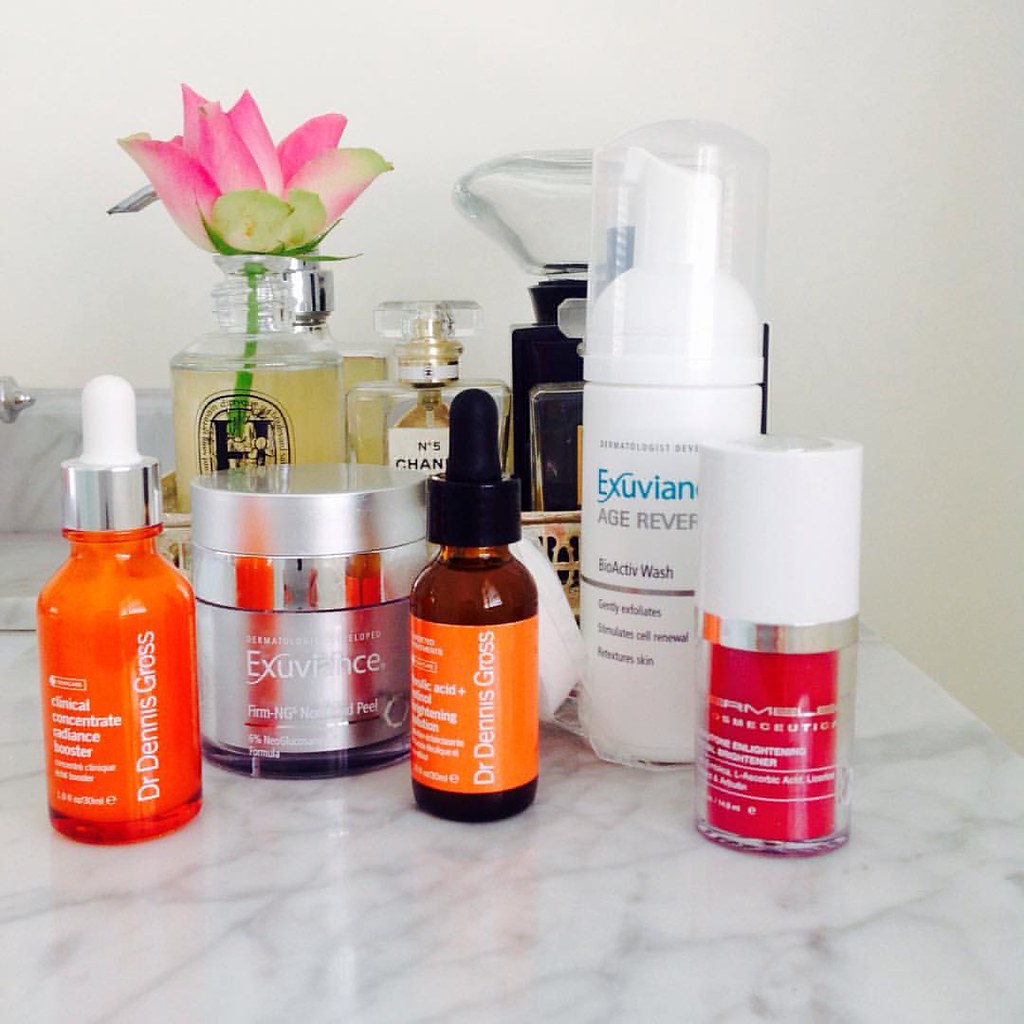This image showcases an array of luxurious cosmetic and skincare products displayed on a pristine marble countertop against a white backdrop. 

In the forefront, two products from Dr. Dennis Gross can be seen prominently: a Clinical Concentrate Radiance Booster in a completely orange bottle with a dropper top, and another product featuring Hyaluronic Acid presented in a brown bottle adorned with an orange label. 

Next to these, the lineup features a Remula Skin Brightening Cream, distinguishable by its striking red bottle capped with a white top and accented with a silver band. Additionally, an Exuviance Age Reverse BioActive product stands proudly, complemented by an Exuviance Firming Peel characterized by its sleek all-silver packaging with white text.

In the background, a classic bottle of Chanel No. 5 makes a sophisticated addition to the collection. Beside it, there is another perfume bottle marked with an 'H,' featuring a delicate flower integrated into its pump, and yet another mysterious black perfume bottle.

The meticulous arrangement of these high-end products against the luxurious marble surface and clean white wall exudes elegance and sophistication.